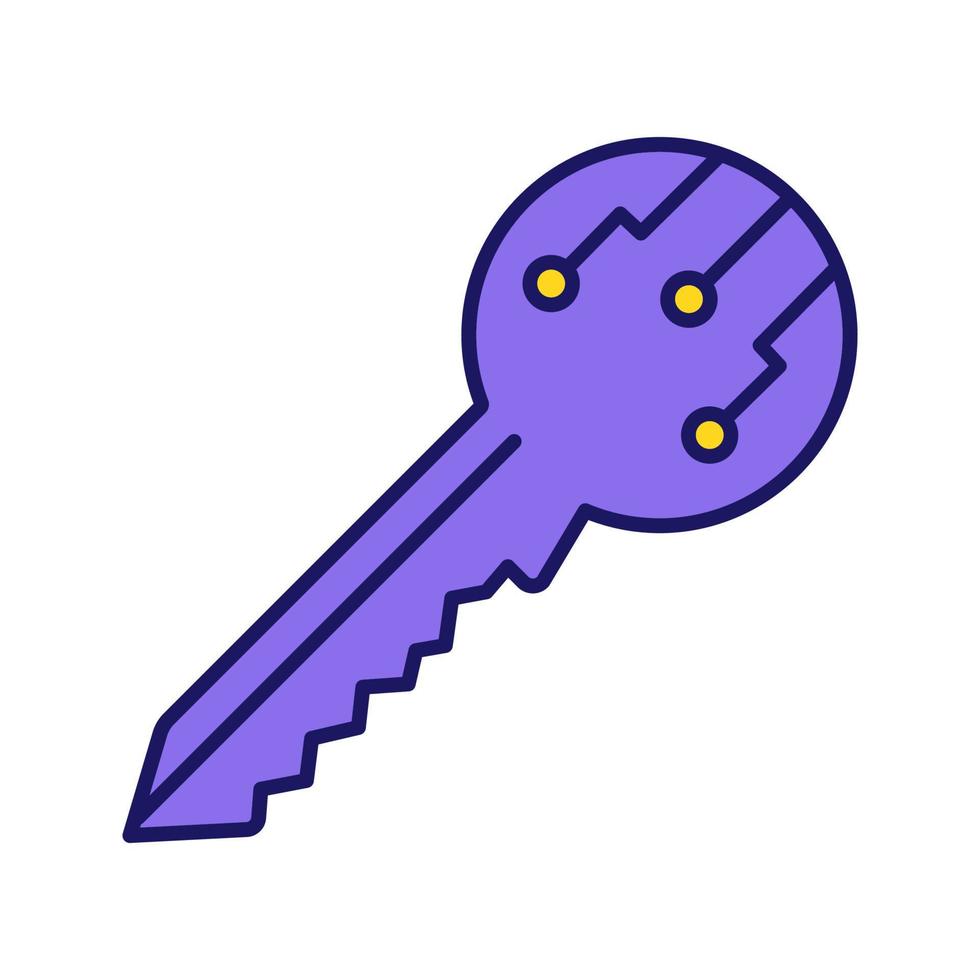This digitally created, color illustration depicts a stylized key with a distinct design. The key has a light purple body with a thin dark blue outline. Its top portion is circular, and the bottom part features jagged edges typical of traditional keys, ending in a pointed tip which is oriented toward the lower left of the image. The circular handle of the key, positioned in the upper right, showcases intricate, circuit board-like projections in dark blue. These projections, resembling microchip runs, extend downward and to the sides, terminating in three symmetrical circles. Each of these circles has a blue outline with a yellow center. A central blue line runs down the length of the key, adding to its dimensionality. The entire illustration stands out against a plain white background.